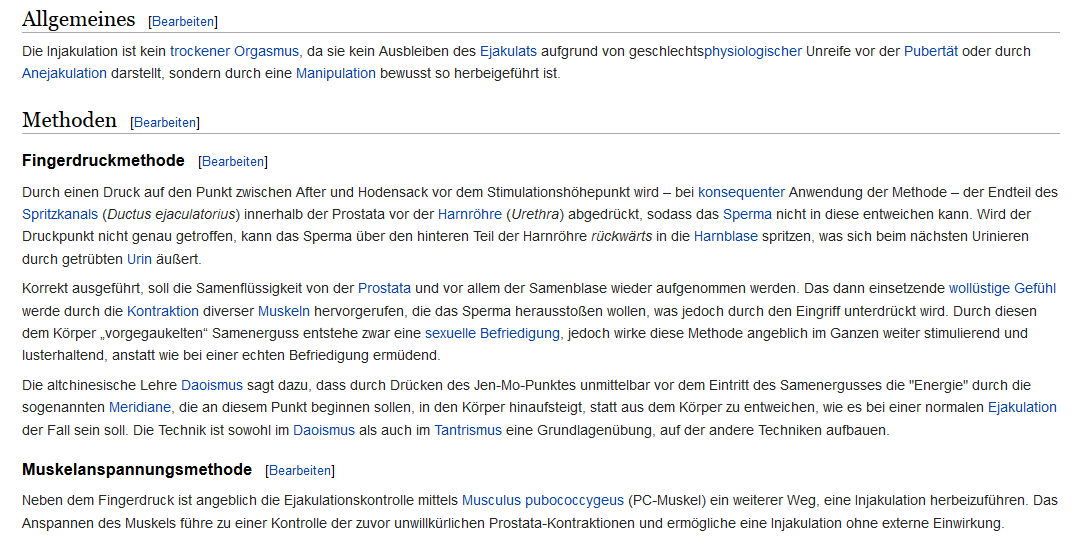The image features a detailed document in a foreign language, resembling a Wikipedia article. The text is predominantly black with some navy blue, and contains multiple sections and hyperlinks in blue. The title at the top is "Allgemeines" written in bold black letters. Below it, another block of text contains the words "die Einjakulation ist kein trockener Orgasmus." 

Further down, a section titled "Methoden" outlines various methods including "Finger der Suck Methode." This section also contains a mix of black text and blue hyperlinks on a white background. At the bottom, another block is titled "Muskelanspannungsmethode," characterized by small black text interspersed with light blue hypertext. The text alignment is predominantly to the left, with certain words emphasized through larger fonts serving as titles.